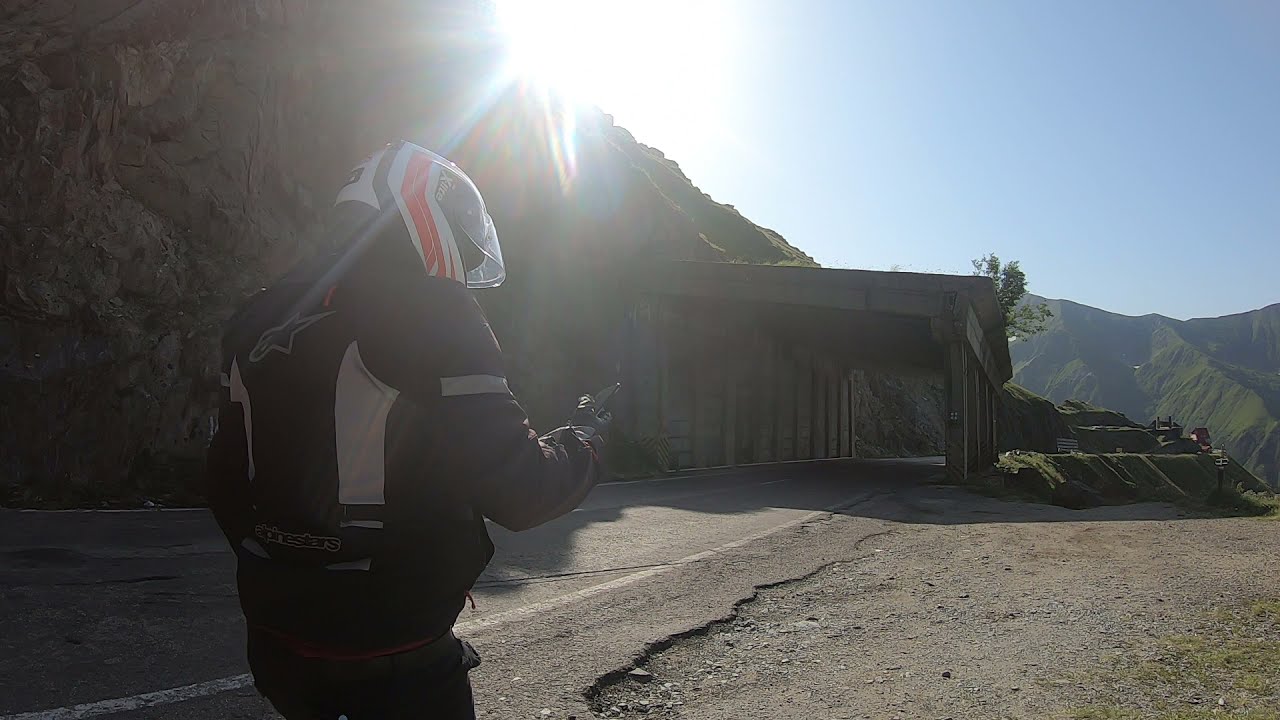A lone figure, dressed in a full black motorcycle outfit, is walking along the dirt shoulder of a deserted two-lane paved road. The individual, whose gender is indeterminate, wears a distinctive helmet that is white, black, and bright orange with a slightly raised visor, obscuring their face as they face away from the camera. The back of their jacket, adorned with a prominent star and "alpine stars" written in lowercase at the bottom, features white patches. Clad in black gloves, they are holding a smartphone and seem to be attempting to make a call. Surrounding them are the dirt and gravel of the road’s edge, beneath an expansive blue sky. The scene is framed by tall mountains and rocks, with an unusual overpass or wooden-structured bridge in the distance that appears to protect the road from potential landslides. This interesting, almost surreal structure adds to the isolated, somewhat desolate atmosphere of the image. A small building and other distant structures can also be seen, highlighting the vast solitude of the landscape.